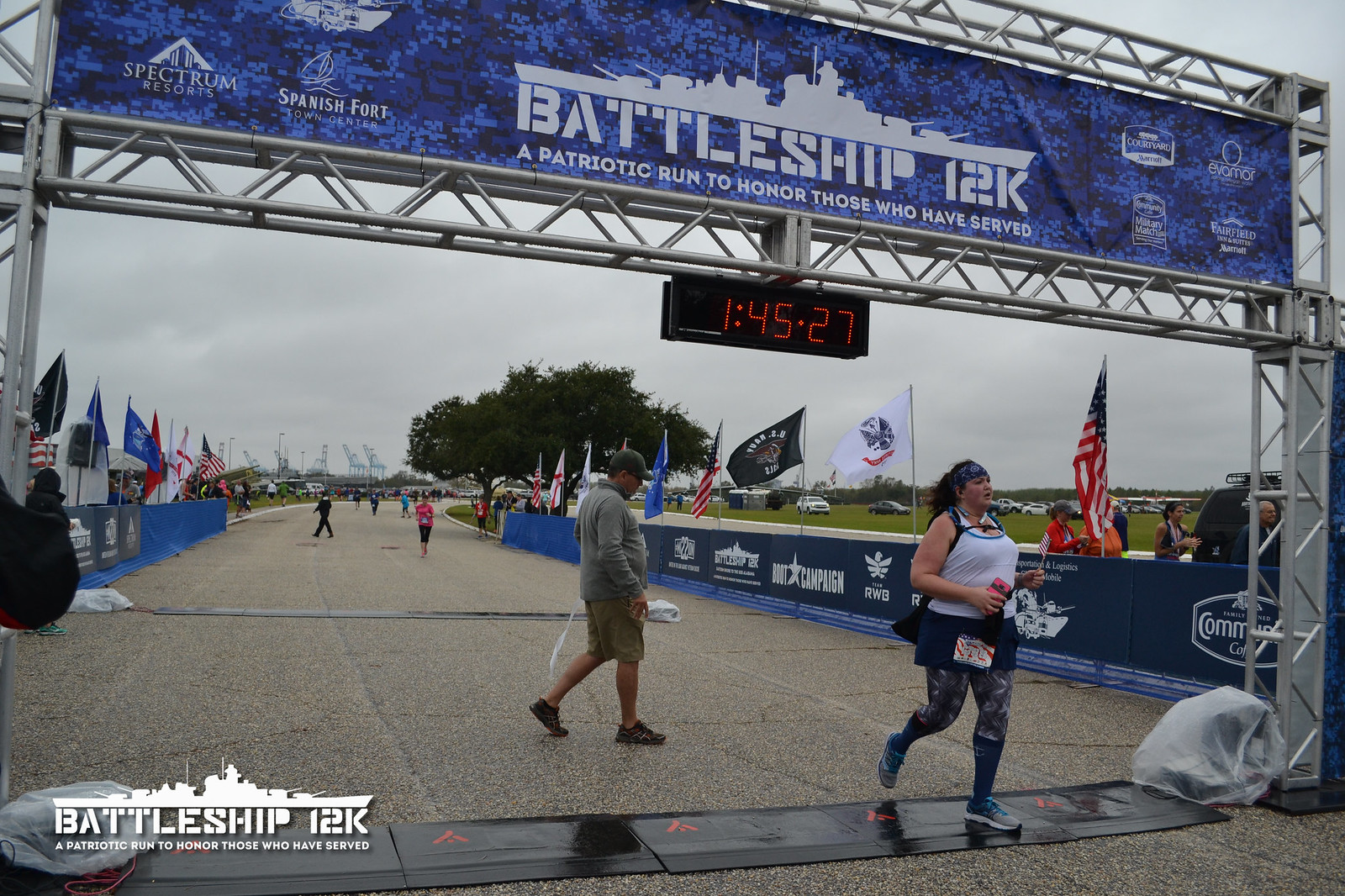In this photograph capturing the finish line of the Battleship 12K, a patriotic run to honor those who served, a robust young woman with blue sneakers, blue knee-high socks, and a white tank top paired with a black running skirt and tights is just crossing the timing mat. Overhead, a big blue banner prominently displays the event's name, "Battleship 12K," and beneath it, the phrase "A patriotic run to honor those who have served" is framed by a silhouette of a battleship. The clock above her shows a finish time of 1 hour, 45 minutes, and 27 seconds. Various sponsor logos are visible on either side of the banner. The surroundings are draped in an array of American flags and other banners, enhancing the patriotic atmosphere. Behind the lead runner, a man in gray walking shorts and a matching sweater walks, seemingly performing a role related to the event. In the distance, additional runners and people can be seen either participating in the race or handling event logistics on this cloudy day. The entire scene is set on an open asphalt area, bordered by barricades adorned with white advertisements.